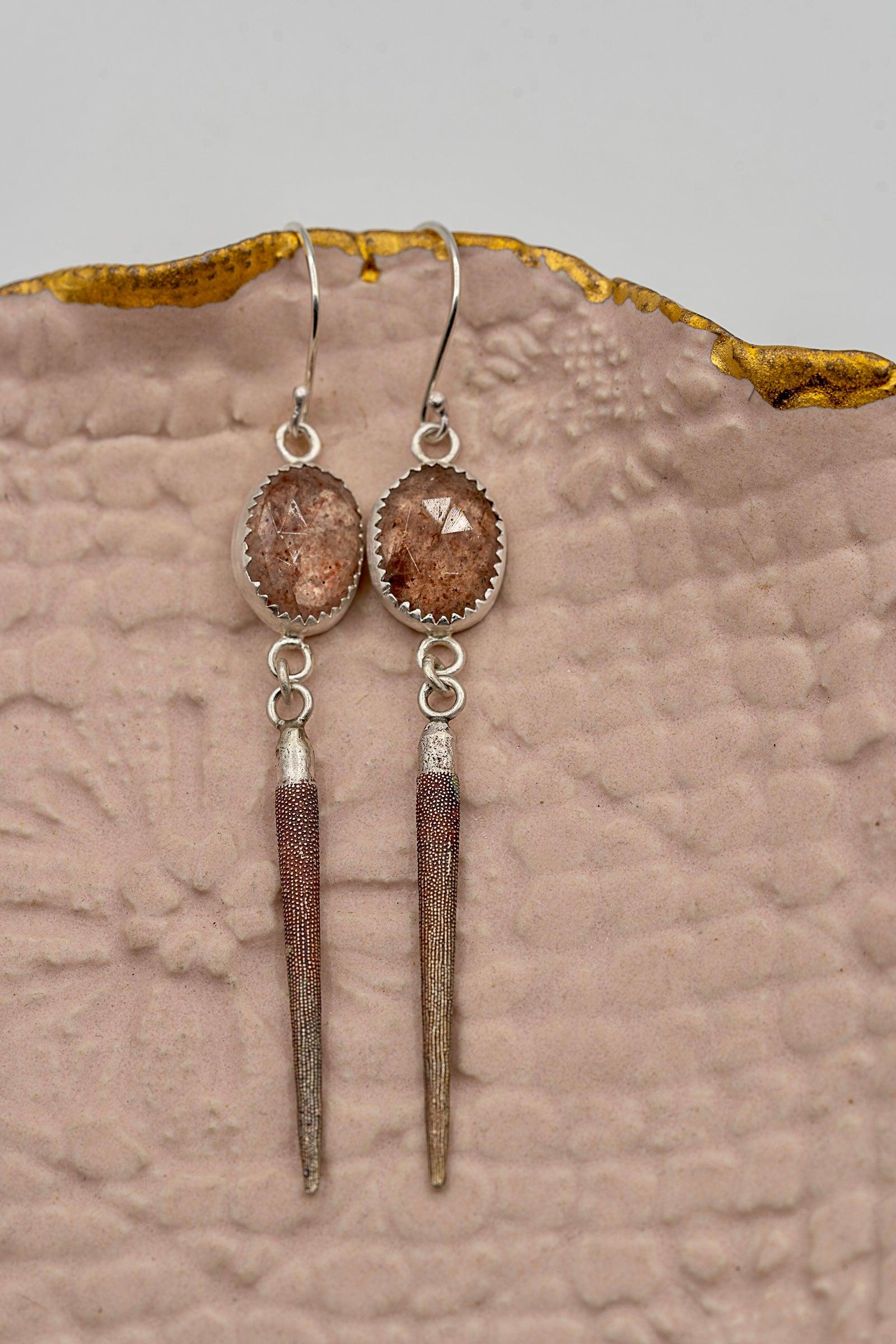The image features a pair of intricate, vintage-style earrings. Each earring showcases a striking, amber-colored gemstone set in a silver frame that resembles a cracked eggshell. This gemstone is delicately spotted, adding a touch of uniqueness. Surrounding the gemstone is a textured silver outer casing. Below this central gemstone, there are two interconnected silver rings, from which dangle long, tapered conical pieces adorned with a series of small, intricate dots, giving them a symmetrical and detailed appearance.

The earrings hang from large, sturdy hooks that are attached to a pink, foam-like display board. This foam has a textured, square pattern and features golden floral designs at the top. The earrings themselves are prominently featured against this backdrop, which adds to the vintage and ornate aesthetic of the jewelry. The setting of the jewelry is gray, providing an elegant contrast that highlights the detailed craftsmanship of the earrings.